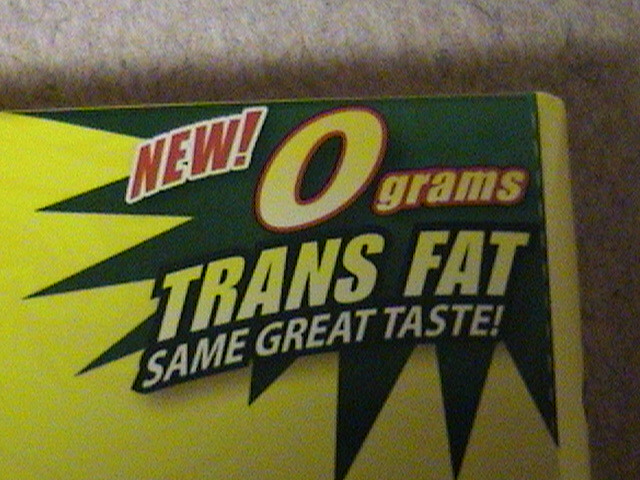This square-shaped image is of low quality, characterized by a blurry and fuzzy appearance due to its low resolution. At the center, partially visible, is a piece of packaging with several notable inscriptions. On the top left, the word "NEW!" is prominently displayed in red with a white border. Adjacent to it, the text reads "Zero grams trans fat," and just below that, it states "Same great taste!" The background features a dark green color with a spiky design pattern, adding texture to the image. Although the image’s clarity is compromised, these textual details and design elements are identifiable.